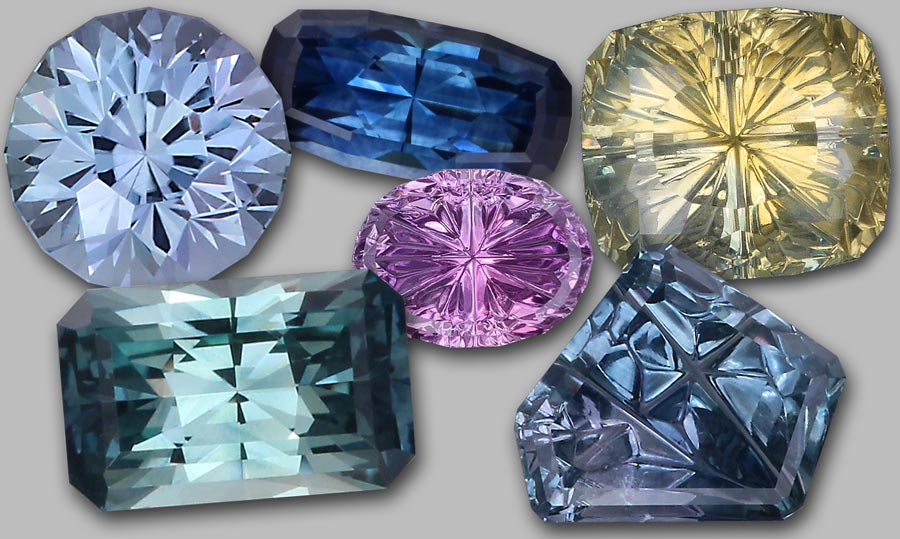This photograph features a meticulously arranged collection of six gemstones, each uniquely cut and displaying a variety of colors and shapes, set against a neutral gray background. The top left gem, reminiscent of a classic diamond cut, is likely a clear or silver diamond. To its right at the top middle, there's an indigo-colored sapphire with a rectangular oval cut. The top right gem has a yellow hue, exhibiting a slightly rounded square cut. In the center of the image is an oval-cut pink amethyst that catches the light beautifully. The bottom row starts with a rectangular-cut emerald on the left, showcasing its vibrant green color. The bottom right features a light blue gemstone with an irregular shape, akin to a pentagon with a side missing, giving it a unique appearance. Each gemstone is brilliantly polished, enhancing their striking colors and sparkling clarity.